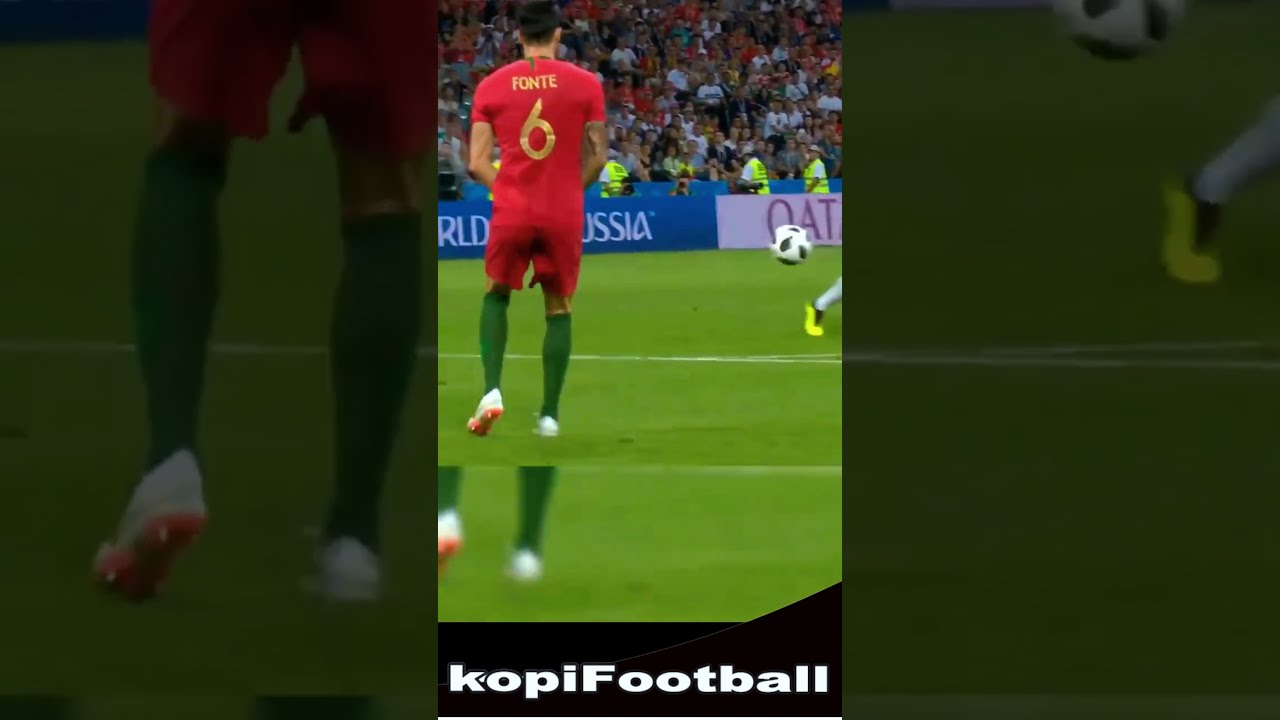The image captures a dynamic moment during a European football (soccer) game. Central to the photo is a single player standing on the left side, facing away from the camera toward a packed stadium. The player, a white male with short dark hair, wears a red uniform comprised of a short-sleeved shirt and shorts, paired with knee-high green socks and white cleats with red soles. His jersey, emblazoned with the name "Fonte" and the number six in yellow letters, stands out vividly against the green pitch.

In the lower right of the image, part of another player's leg and foot is visible next to a soccer ball patterned with black and white markings, seemingly in motion. The crowd in the background is dense, with spectators filling the stands and security personnel in neon yellow vests stationed along the perimeter. 

The scene is filled with a spectrum of colors, including the green of the field, various skin tones, and the vibrant hues of the players' uniforms and the audience's clothing. Additionally, some text with characters like R, O, D, U, S, S, I, A, Q, and T can be seen on a banner in the background, perhaps indicating a larger event or location reference. At the very bottom of the image, a caption in white text on a black background reads "Kopi Football."